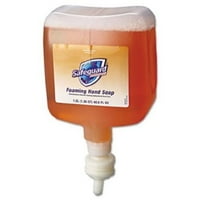The image is a photograph of a large, industrial-sized bottle of Safeguard antibacterial foaming hand soap. The bottle is placed upside down, with the white cap and circular dispenser at the bottom. The container itself is a rectangular box shape, made of clear plastic, allowing the mostly full orange liquid soap inside to be visible, along with some bubbles concentrated near the cap. The label on the front features a blue badge with a white trim that reads "Safeguard," and below it states "Foaming Hand Soap" along with the volume measurements of 1.2 liters (1.25 quarts or 40.5 fluid ounces). The overall background of the photograph is solid white, making the soap bottle appear to be floating in a white void. No hands or other objects are holding the bottle, giving it a clean, product-focused presentation.